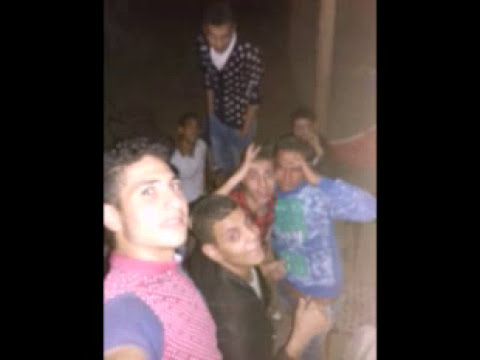In this dimly lit indoor setting, seemingly a party or gathering, the photograph captures seven young men, arranged within a square image framed by black borders on the left and right sides. Central to the image, and positioned in the bottom left corner, a man with black curly hair and subtle sideburns wears a pink shirt with blue short sleeves. He is taking a selfie, his face reflecting a look of shock or fear, as he gazes towards the right.

Next to him, another man with a darker complexion and black hair, dressed in a black long-sleeve jacket over a white shirt, also looks towards the right. Behind these two, a pair of guys are closely posing with their faces touching; the one on the left sports a red shirt and raises his right hand in a playful gesture, while the other, in a blue shirt with green spots, mirrors the intimacy.

In the background, slightly out of focus, a man in a black shirt oversees the scene, further highlighted by a taller figure elevated above the rest, wearing a black shirt with white dots and blue jeans. Lastly, to the far left, another man in a short-sleeve white shirt completes the group, all encapsulated within a dark, somewhat chaotic room. The image captures their spontaneous and candid expressions, illuminated faintly by ambient lighting.